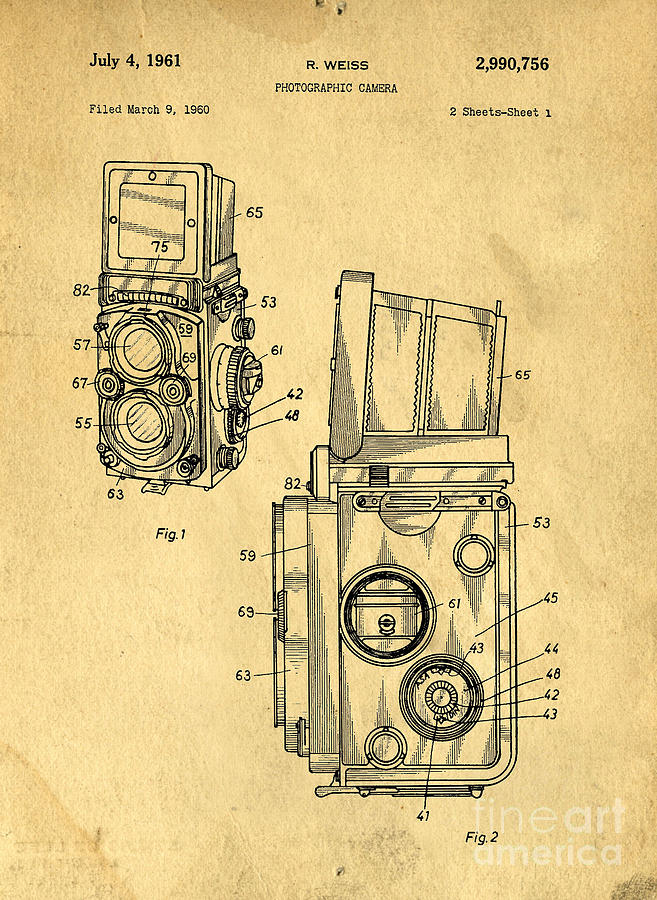This is an elaborate instructional diagram of a vintage camera, showcased through two views: one from the side and one from the front. Each part of the camera is meticulously labeled with numbers pointing to various sections, illustrating the mechanical intricacies of the device. The diagram, etched in black ink, is set against a yellow, slightly browned paper that evokes an antique feel. 

In the top left corner, there is text noting the dates "July 4th, 1961" and "Filed March 9th, 1960," along with the name "R. Weiss" and the term "Photographic Camera." Additionally, the patent number "2,990,756" is prominently displayed. A faint white watermark at the bottom right reads "Fine Art America," indicating the probable distributor of this poster. The entire piece exudes a historical essence, suggesting it could be a reprint or representation of the original patent drawing filed for a patent on the specified dates.